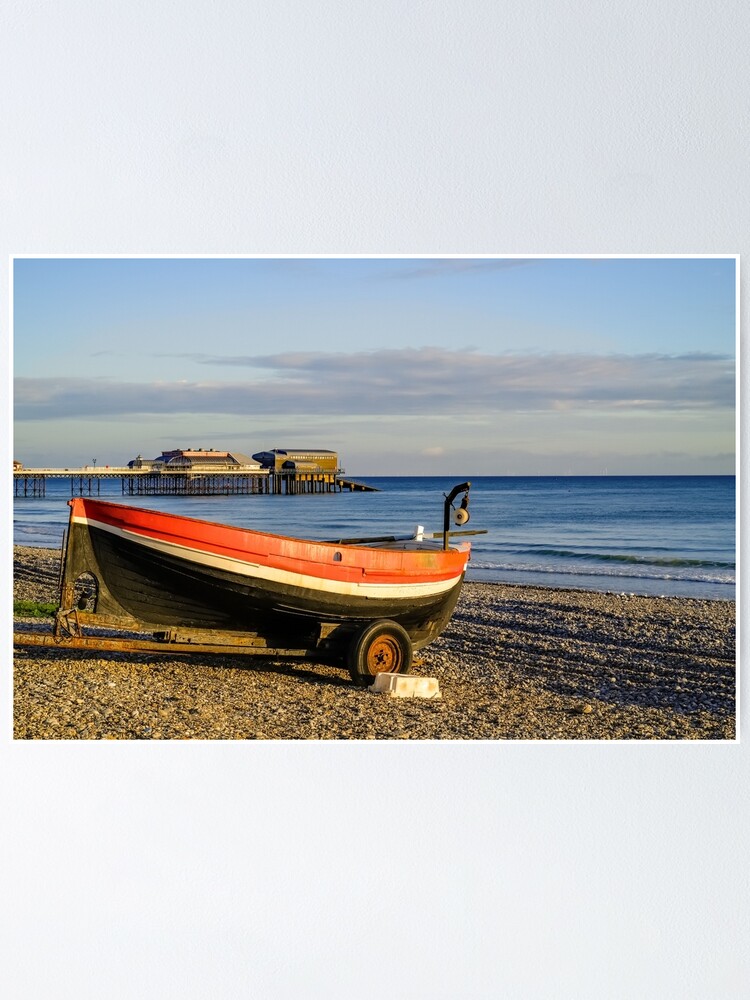The image showcases a small, wooden boat designed for two people, featuring a crank mechanism at the back, likely used for pulling something out of the water. The boat's hull is black with a white stripe and red on top. An oar is visible inside the boat, which is situated on an old, rusty trailer with a cement block by the tire to prevent it from rolling. The boat is backed up to the edge of a coarse gravel shoreline, in front of calm, bright blue water under a light blue sky with a few clouds. In the distance, a large pier extends into the water, with two buildings and a ramp leading down to the water. The pier is supported by posts and includes a walkway for people. The overall scene suggests a tranquil, outdoor coastal environment ready for boating activities.